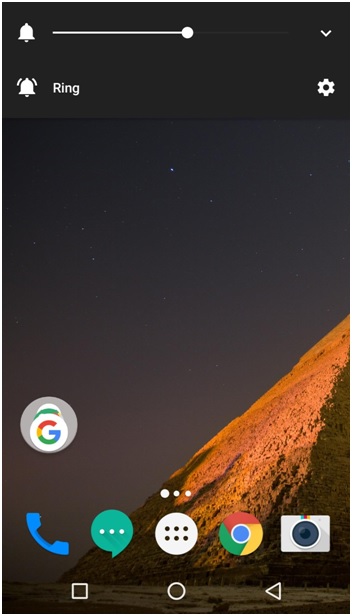Screenshot of an Android Phone Homepage

At the very top of the image, a black opaque box displays the user adjusting the notification volume. Inside the box, on the left, there's a white bell icon followed by a white slider bar set just past the halfway mark. On the right side of the slider is a downward arrow. Beneath the slider and the initial bell icon, another white bell icon appears, this one with ringing lines indicating sound. To the right of this second bell icon is the small white text "Ring." On the far right of this section, there's a settings button.

The main part of the screen is dominated by the phone's home screen background, which features a stunning night sky and a pyramid. The pyramid, located at the bottom right corner of the background, reflects a sunset, casting a visible shadow. Above the pyramid, the sky transitions from a faded orange near the horizon to deep black, dotted with stars.

Located at the lowest part of the screen are several app icons. From left to right, these include a phone icon, a message icon, a Chrome browser icon, and a camera icon. In the middle of these icons is a circle with six smaller circles inside, likely representing the app drawer. Beneath these icons are the phone's navigation buttons: the recent apps button (depicted by a square), the home button (depicted by a circle), and the back button (depicted by a triangle).